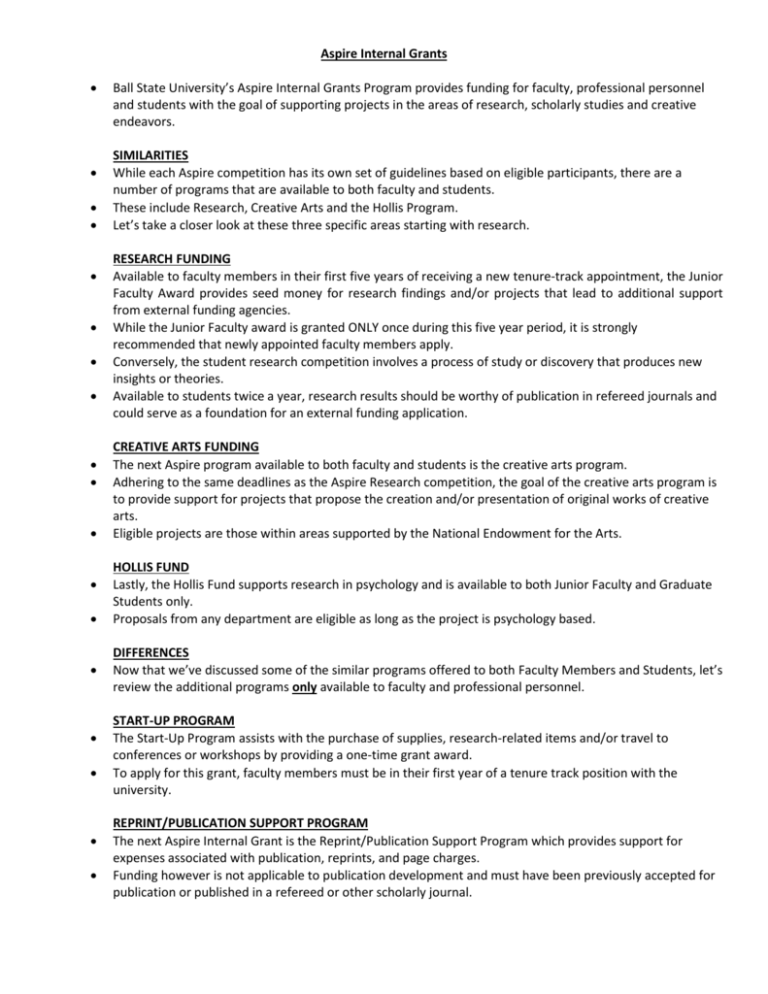This image, titled "Aspire Internal Grants," features an announcement from Ball State University highlighting its Aspire Internal Grants Program. The program aims to provide funding to faculty, professional personnel, and students to support a variety of projects, including research, scholarly studies, and creative endeavors. The information is presented in a clear, bullet-pointed format, with key sections highlighted in bold and underlined for emphasis.

At the top, the caption outlines the purpose of the Aspire Internal Grants Program. The following bullet points summarize the similarities and differences in the types of funding available:

**Similarities:**
- **Research Funding**
- **Creative Arts Funding**
- **Hollis Fund**

**Differences:**
- **Startup Program**
- **Reprint Publication Support Program**

The caption further explains that, after discussing the similar programs available to both faculty and students, there is a section dedicated to additional programs that are exclusively offered to faculty and professional personnel. These distinctions highlight the tailored support provided by Ball State University to cater to the varied needs of its academic community.